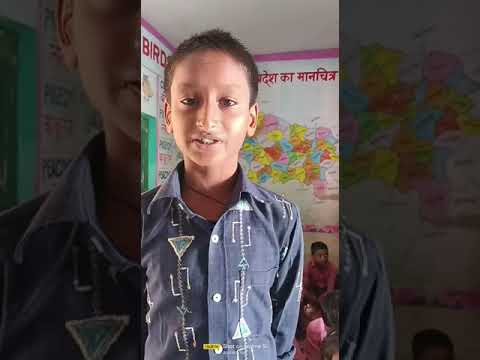The image showcases a young boy standing in what appears to be a classroom setting. The photo, taken in vertical portrait mode, features darkened bars on either side typical of this format. The boy has very short brown hair and wears a dark blue, button-down long-sleeved shirt adorned with white designs. The shirt's pattern includes triangles pointing up and down, dotted lines, and square-like formations. Additionally, he has a necklace, though its details are unclear. Behind him, a colorful world map is visible, displaying hues of yellow, orange, and blue. The top left corner of the wall features the word "birds" in red English letters, while other writing in a foreign language, possibly Hindi, appears above the map. The background is part of a larger faded image, framing the main vertical portrait. The boy looks directly into the camera, capturing a candid moment in what looks to be an educational environment.